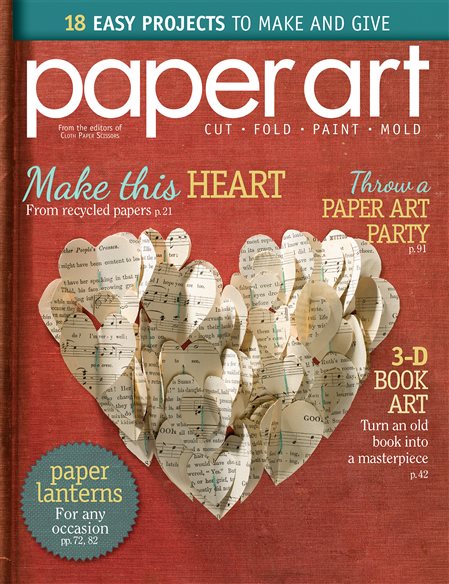This image showcases a vibrant magazine cover designed with a warm, orangey-red background. Dominating the top banner, set against a turquoise background, is the bold headline in white and yellow text: "18 Easy Projects to Make and Give." Below this announcement, the title "Paper Art" is prominently displayed in large white letters, followed by the smaller text, "Cut, Fold, Paint, Mold." Central to the cover is an intricate heart composed of layered and recycled paper hearts, many featuring text from poems or old music notes, meticulously shaped into a larger heart. The magazine tempts creativity with enticing project highlights such as "Make this Heart from Recycled Papers," "Throw a Paper Art Party," "3D Book Art: Turn an Old Book into a Masterpiece," and "Paper Lanterns for Any Occasion," complete with page references. This captivating cover serves not only to inspire but also directs readers to Beadaholique.com for all their beading supply needs.